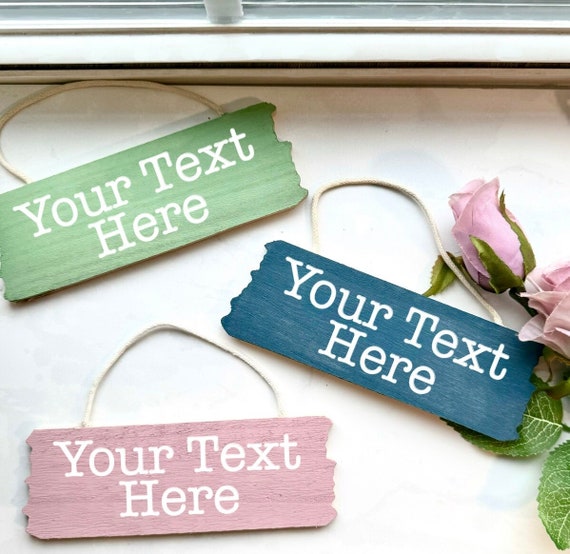The square image features a beige tray with a raised edge, set against a window backdrop, identifiable by the horizontal white strip at the top and a glimpse of the window pane. On the tray, there are three rectangular signs with uneven edges, each painted a different color and inscribed with "your text here" in white letters. The signs, which have thin light brown ropes attached for hanging, include a green sign in the upper left, a blue sign in the middle, and a pink sign at the bottom. Adding a touch of nature, a light purple flower with green leaves lies on the right side of the tray.